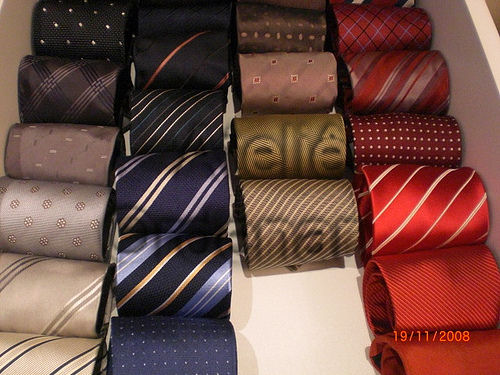This photograph, stamped with the date 19/11/2008 in the bottom right-hand corner and bearing an artist watermark that reads "ELIE DRANAN," showcases a meticulously organized drawer filled with rolled-up ties, neatly arranged by color. The first column on the left features ties in black, gray, silver, and beige hues, including a black tie with white dots, a black tie with gold stripes, a gray tie with gold flecks, a silver tie with floral patterns, and a beige tie with gold stripes. The second column is predominated by blue ties of various patterns, such as stripes and dots. The third column displays a collection of brown ties, although it contains fewer ties than the other columns. The final column on the right features ties in various shades of red, showcasing patterns ranging from plaid to polka dots. Each tie within the drawer carries a distinctive pattern, encapsulating a diverse range of designs from simple solid colors to intricate stripes and dots.